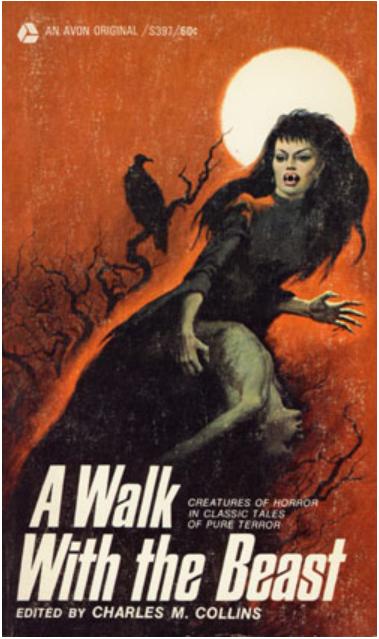This image is a vintage book cover for an Avon original publication priced at 60 cents. The top of the cover features the text “An Avon Original” along with a small recycling symbol. The title, prominently displayed at the bottom in small white text, reads "A Walk with the Beast," and beneath it, "Creatures of Horror and Classic Tales of Pure Terror," edited by Charles M. Collins.

The background of the cover is a striking red with an eerie full moon, casting an ominous glow over the setting. Shadowy, creepy trees with sparse leaves frame the scene, with a vulture perched menacingly on a branch. Dominating the scene is a vampiric woman with sharp fangs, long black hair, and heavy makeup, including red lipstick. She is dressed in a long, black dress and appears to be carrying a small, seemingly lifeless young boy in her arms. The scene suggests a chilling narrative, encapsulating elements of pure terror and classic horror.